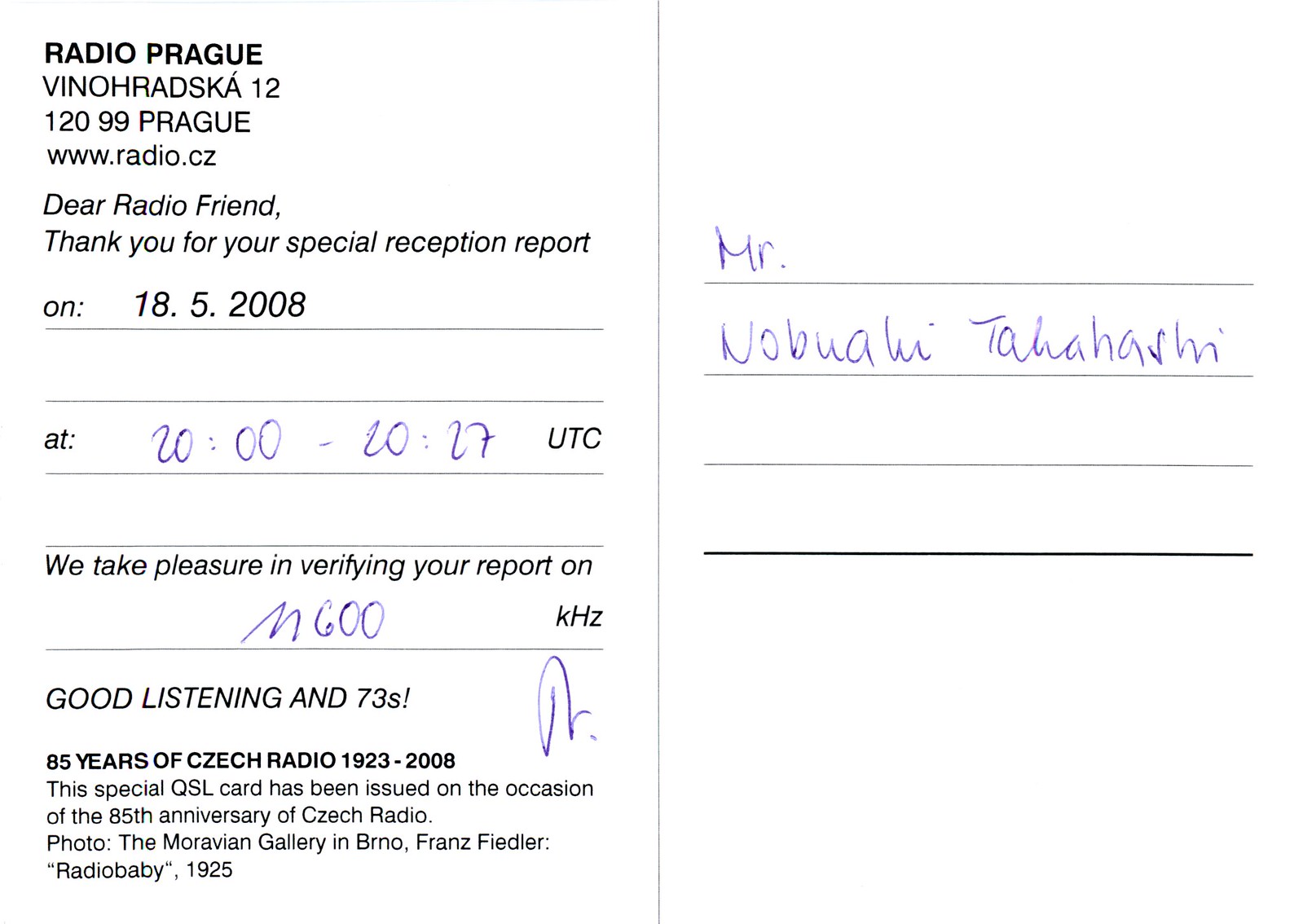The image depicts a simple print piece with a white background featuring black printed text and blue handwritten notes. At the top left corner, it prominently says "Radio Prague." Below that, an address and a website are printed. Further down, the text reads, "Dear Radio Friend, Thank you for your special reception report on 18.5.2008." Handwritten in blue ink, the time "21:20:00 hours to 20:17 hours" is noted. The text continues, "We take pleasure in verifying your report on M600 K kilohertz. Good listening and 73." On the other side, in handwritten blue ink, the recipient's name appears as Mr. N. Obua, with the first name Tanahashi written below. Additional handwritten and printed details mention phrases like "85 years of tech radio" and "special QXL Spark," along with references to Studio Kona, Mojave, Galloway, and Reno. The handwritten aspects suggest a personalized touch, filling in specific details to complete the postcard.